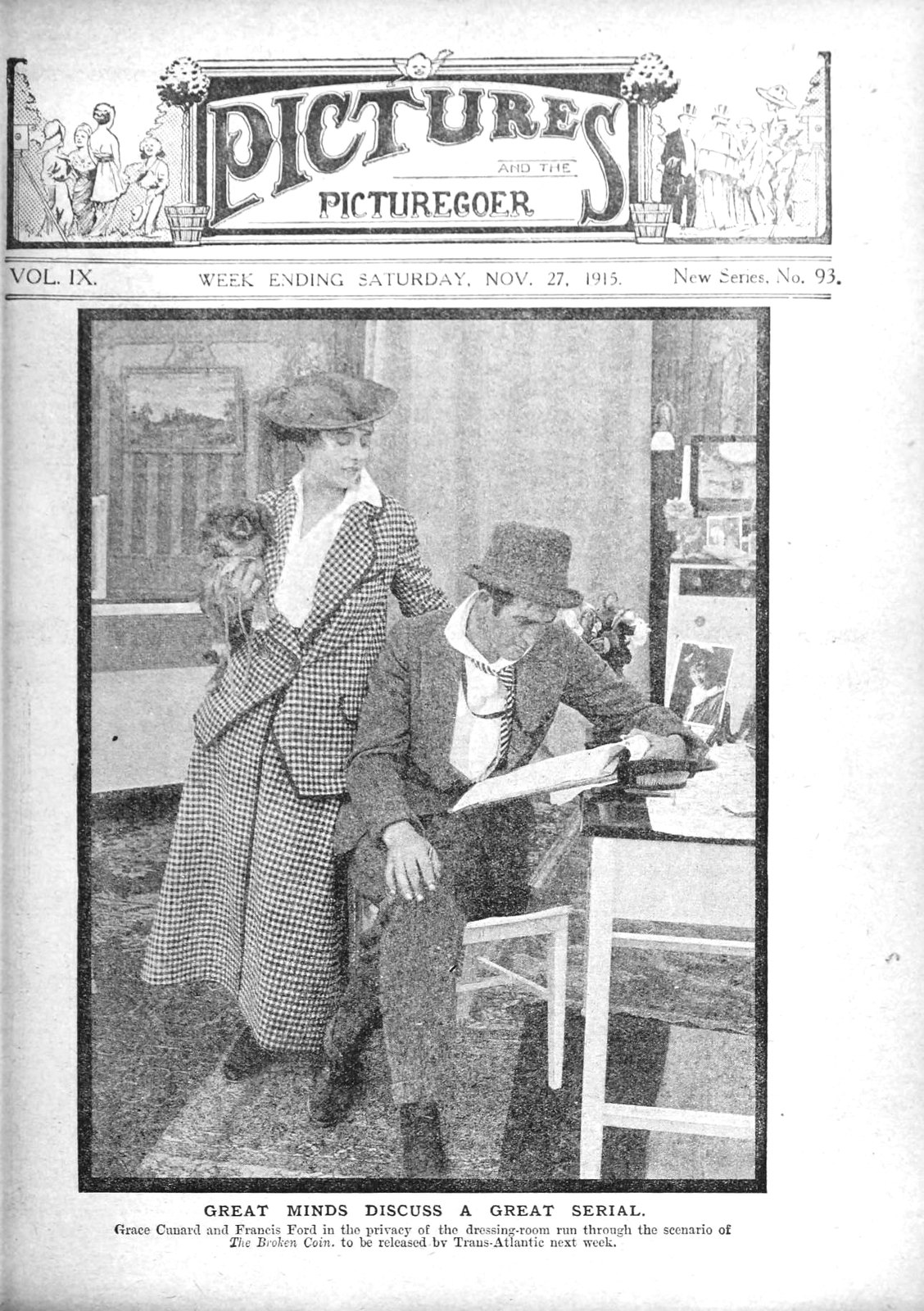This vertical, rectangular image depicts the cover of a vintage magazine titled "Pictures and the Picture Goer." The issue is identified as Volume IX, New Series Number 93, for the week ending Saturday, November 27, 1915. The heading and title of the magazine are prominently displayed at the top, encased in a decorative frame. Below the heading, a faded black-and-white photograph shows Grace Cunard and Francis Ford, renowned individuals of their time, as they appear to discuss the scenario for "The Broken Coin," scheduled for release by Transatlantic the following week.

In this photograph, Grace Cunard is seen standing, dressed in a long skirt and a matching coat, with a flat hat perched on her head. She is holding a small dog in her right arm and is looking down over the shoulder of Francis Ford. Ford, meanwhile, is seated at what seems to be a dressing room table, adorned with various items including a bouquet of flowers and framed photos. He is reading a script, appearing engrossed, with his attire consisting of a disheveled tie, an open coat, a matching color suit, and a round top hat. At the bottom of the image, the caption reads, "Great Minds Discuss a Great Cereal," providing context to the intimate and focused nature of the photograph.